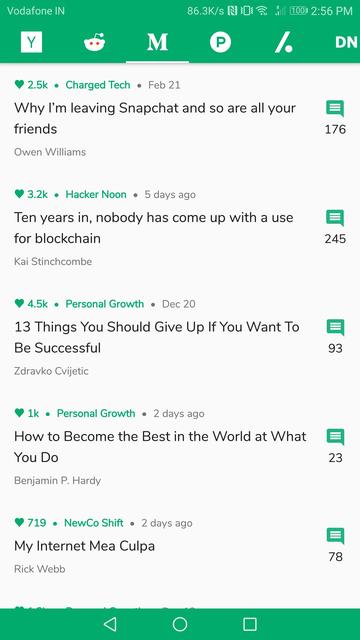The image is a screenshot from a cell phone. At the top, there is a wide green horizontal rectangle spanning the width of the screen. In the upper left-hand corner, the word "Vodafone" is displayed in white. In the center and extending to the right are white status icons, including the battery level, time, and cellular reception signal.

Below this top bar, a row of app icons is visible:
1. A white square featuring a black "Y."
2. The Reddit mascot icon.
3. A capital white "M."
4. A white circle containing a green "P."
5. An icon resembling a slash with a period on the right side.
6. At the far right, a capital "DN" in white.

Beneath the app icons, several rectangular notification bars are displayed with text summaries and interaction counts:
1. "Why I'm leaving Snapchat and so are all your friends" with a green square message icon beside it and the number 176.
2. "10 years in, nobody has come up with a use for blockchain" with a green message square indicating the number 245.
3. "13 things you should give up if you want to be successful" with an interaction count of 93.
4. "How to become the best in the world at what you do" with the number 23.
5. "My internet mea culpa" accompanied by the number 78.

At the very bottom, there is a horizontally-aligned green rectangle. In the center of this rectangle is a white-outlined circle. To the left of the circle, there is an arrow symbol, depicted as a sideways triangle pointing left. To the right of the circle is a square icon.

This detailed description covers all visible elements and respective information in the screenshot.